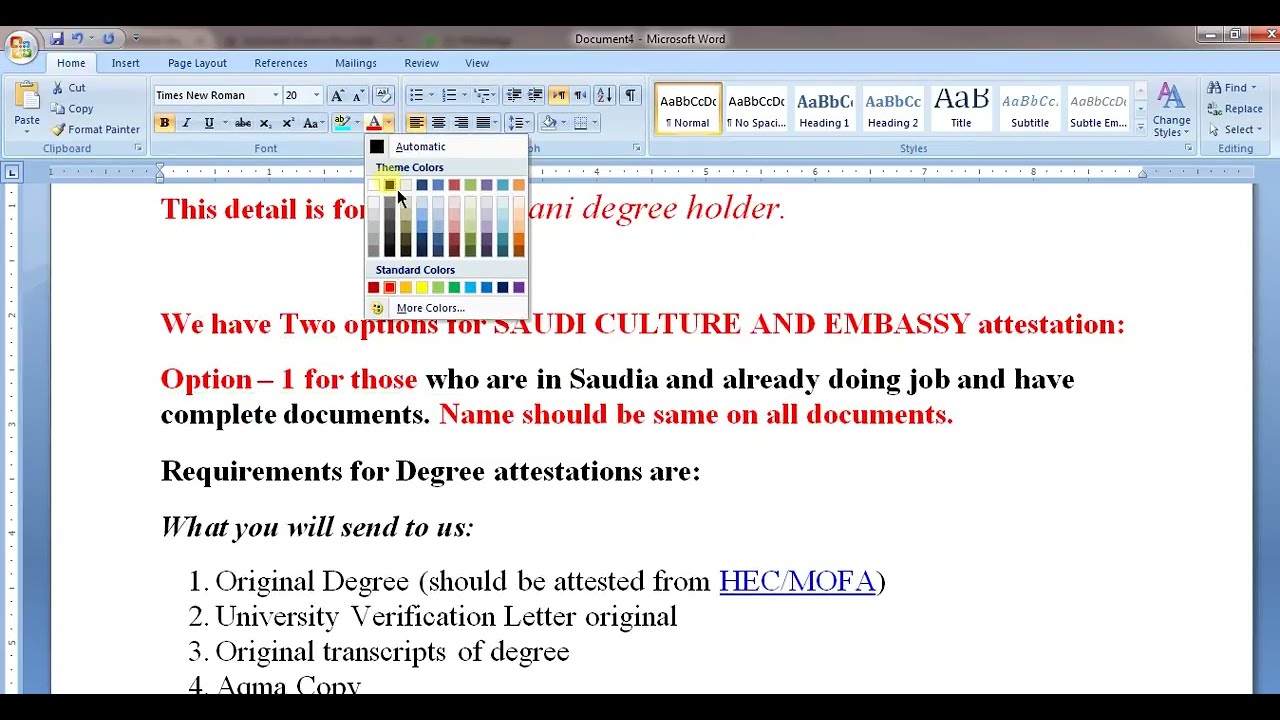The screenshot displays a Microsoft Word document on a computer screen, characterized by a familiar toolbar at the top in a light blue shade. The cursor has opened the font color selection icon, resulting in a small pop-up box displaying a grid of different colors, partially covering the text below. The section directly below the toolbar is the main body of the document, featuring text in various colors. In red text at the top, it reads, "The detail is for a blank degree holder." Subsequently, it mentions, "We have two options for Saudi culture and embassy attestation," also in red. 

Switching to black, it outlines that Option one is for individuals in Saudi Arabia who are already employed and possess complete documents, highlighting that names must be identical on all documents. Transitioning back to red, another crucial detail is emphasized. Below this, the document reveals a list of requirements in black font:

1. The original degree must be attested by the HEC and MOFA.
2. An original university verification letter.
3. Original transcripts of the degree.
4. An AOMA copy (partially obscured).

The white document stretches underneath this text, displaying a typical view of a Word page, indicating detailed information crucial for degree attestation processes.